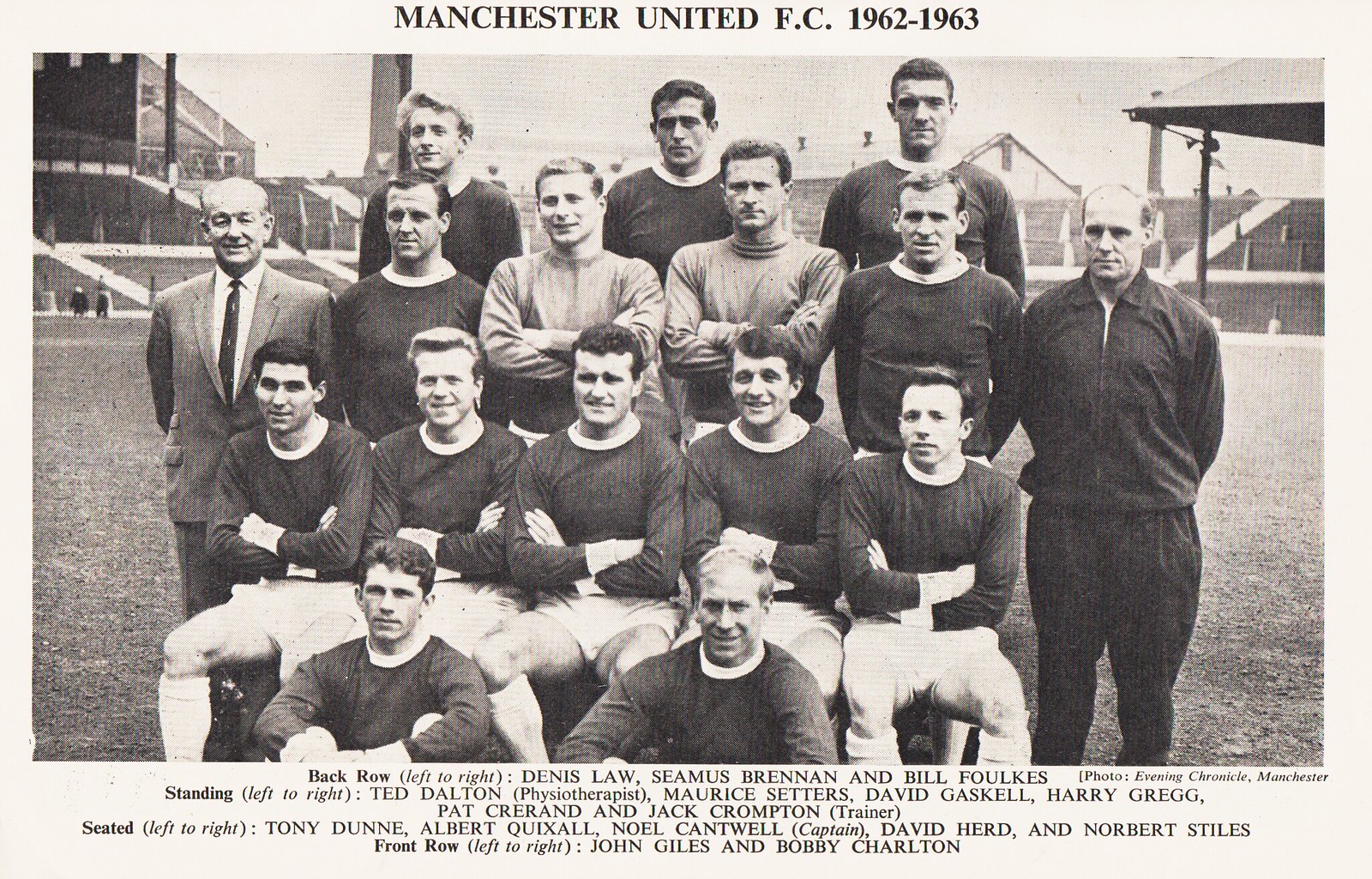This black-and-white photograph captures the 1962-63 Manchester United F.C. team in a meticulously structured formation. Positioned against a backdrop of bleachers, the team consists of 16 members dressed in long-sleeve uniforms, indicative of a chilly day in Manchester. The image is framed with a white border, bearing the caption “MANCHESTER UNITED FC 1962-1963” at the top and detailed player identifications at the bottom. Arranged in four rows, the front row includes John Giles and Bobby Charlton seated on the ground. Directly behind them, seated from left to right on chairs are Tony Dunn, Albert Quicksall, Captain Noel Cantwell, David Hurd, and Norbert Stiles. The third row features players standing from left to right: Dennis Law, Seamus Brennan, Bill Foulkes, physiotherapist Ted Dalton, Maurice Setters, David Gaskell, Harry Gregg, and Jack Crompton. In the back row, also standing, are three taller men: Dennis Law, Seamus Brennan, and Bill Foulkes. This photograph not only highlights the team's composition but also their support staff, emphasizing a well-rounded, robust squad from that historic season.